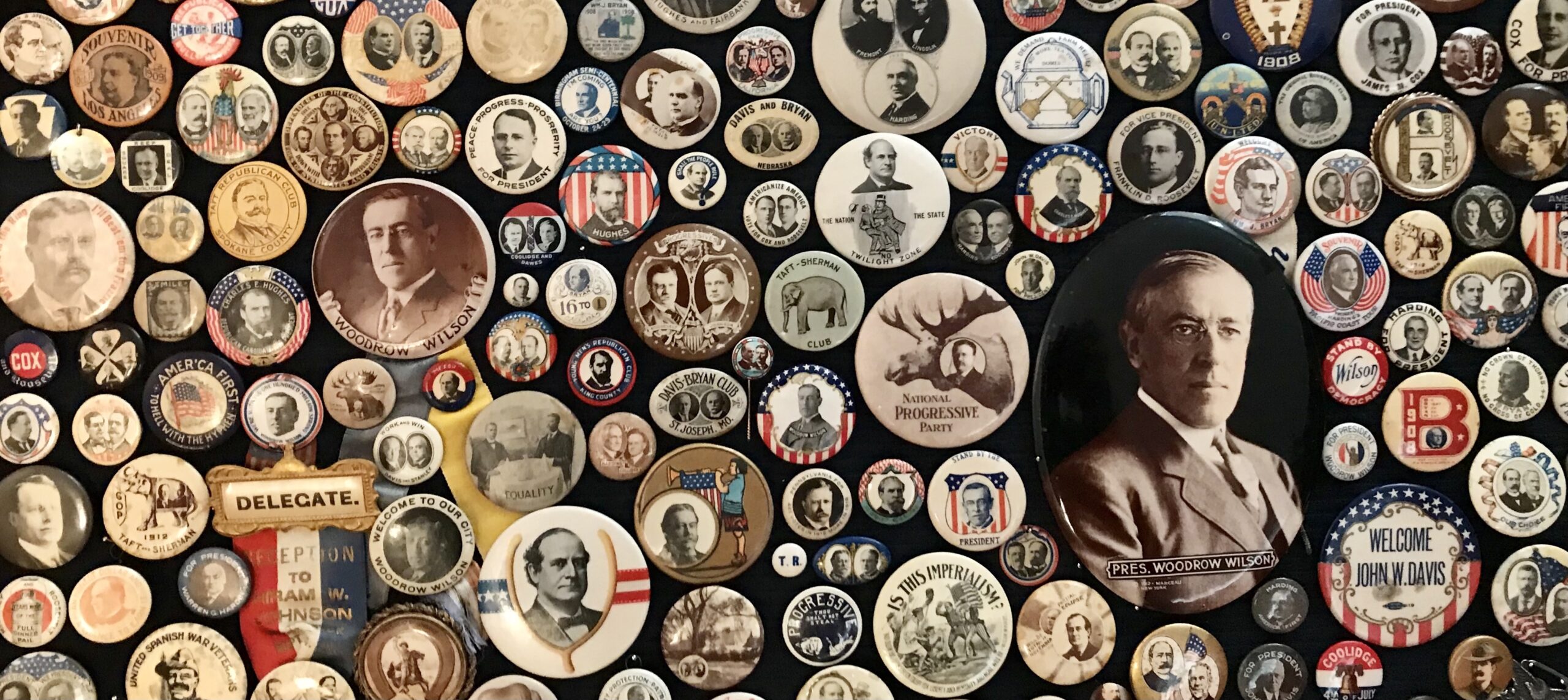The image depicts an extensive collection of U.S. political campaign buttons, spanning multiple elections and featuring various delegates and presidents. Among the more prominent buttons are one with a large portrait of President Woodrow Wilson, showcasing him in a brown suit against a black background. Adjacent to this is a vibrant red, white, and blue button welcoming John W. Davis, with a circular design where the blue field with stars meets the striped section. Another notable button displays Teddy Roosevelt's face superimposed on a moose, labeled "National Progressive Party," emphasizing its vintage appeal. The collection also includes a button with an elephant symbol, various buttons depicting different white male political figures, and a red, white, and blue "delegate reception" pin, although the name on it is unclear. In total, there appear to be about a hundred buttons of varying sizes, from very small campaign pins to larger, almost portrait-like buttons. A small button possibly depicting Queen Elizabeth is also visible at the top left. Some buttons are too small to discern specific details, but the collection overall offers a rich visual history of U.S. political memorabilia.